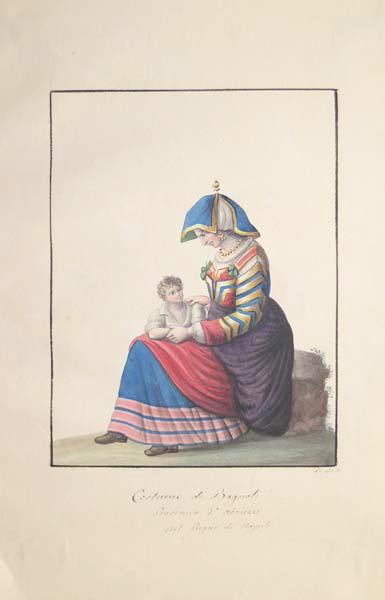This painting features a detailed illustration of a woman sitting gracefully on a large rock on a concrete floor. The image is framed by a bold black rectangle with three faint lines of text below the picture, too faded to read clearly. The woman, adorned in an elaborate, multi-layered dress, appears to be a mother gazing down at a small child seated in her lap. 

Her dress is a composition of rich colors and intricate patterns: the upper portion alternates between stripes of blue and gold, while the shoulders and wrists are accented with red and white details. The lower part of her dress includes blue and pink striped layers, with an overlay of reddish-burgundy fabric on her knees and a purple apron-like cloth draped around her waist. 

A notable feature is her unique head covering, resembling a cloth umbrella trimmed in gold, with an underlying white layer and a small spire crown on top. She also wears a golden necklace, adding to her regal appearance. 

The child on her lap has curly brown hair and is dressed in simple white clothing. The baby, though small, is depicted with notable definition, suggesting a muscular form. The scene is bathed in earthy tones, predominantly browns and tans, creating a serene and timeless atmosphere.